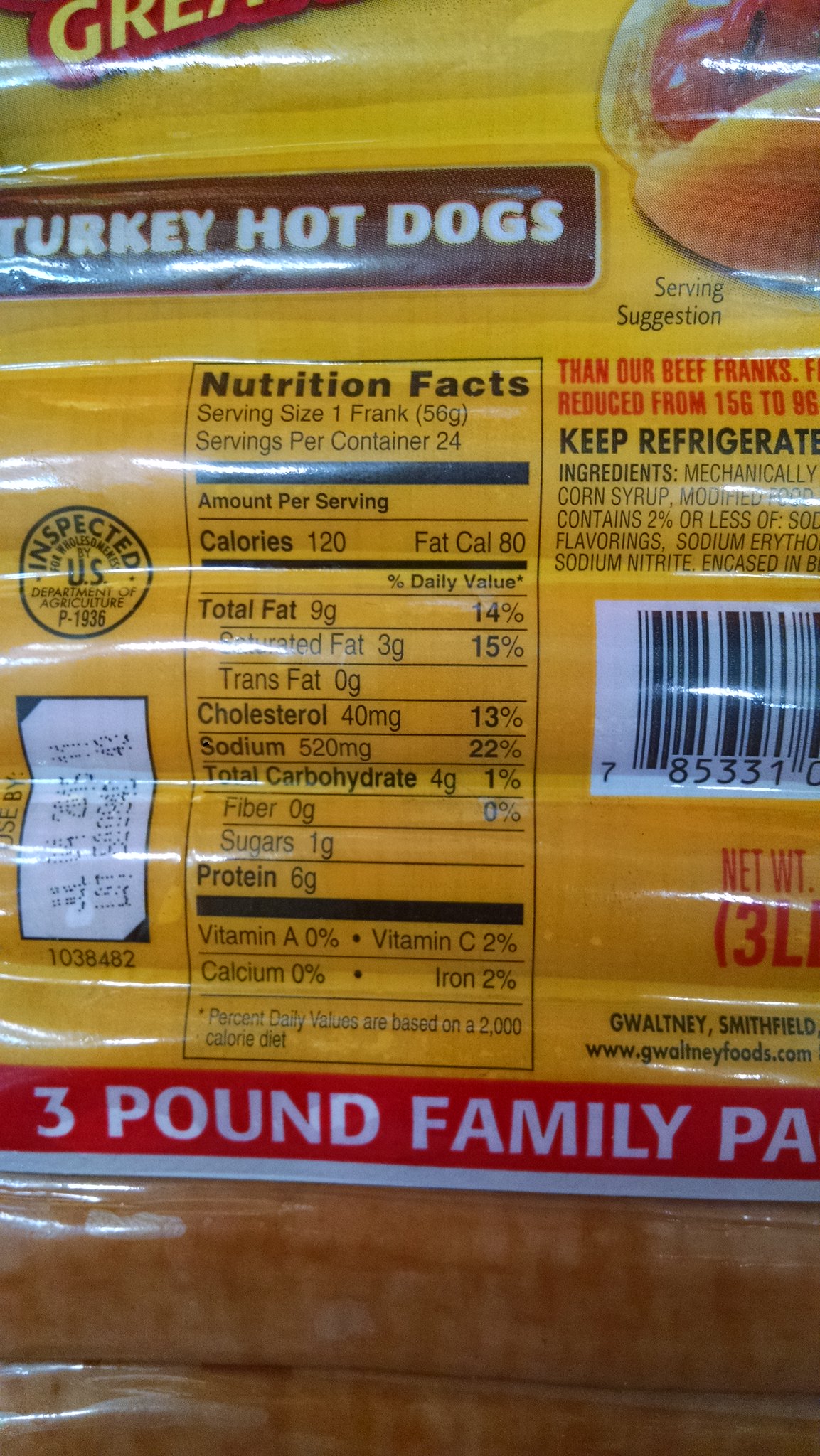The image depicts the back of a yellow and red packaged family pack of turkey hot dogs, specifically a 3-pound package. The top of the package features a brown square where "Turkey Hot Dogs" is prominently displayed in white text. Adjacent to the text is a partial image of a turkey hot dog nestled in a bun. The detailed nutrition facts panel indicates a serving size of one frank, with 24 servings per container. Each serving contains 120 calories, 9 grams of fat, 40 milligrams of cholesterol, 6 grams of protein, and 4 grams of total carbohydrates. 

Additionally, a small circle inscribed with "Inspected U.S." and the number "P-1936" implies USDA inspection. There's also a clear instruction to keep the product refrigerated. Partial ingredients are visible on the package, as well as a barcode with the numbers "853310" and an additional "7" off to the side. At the bottom of the package, the designation "3 Pound Family Pack" is displayed in bold red and white lettering.